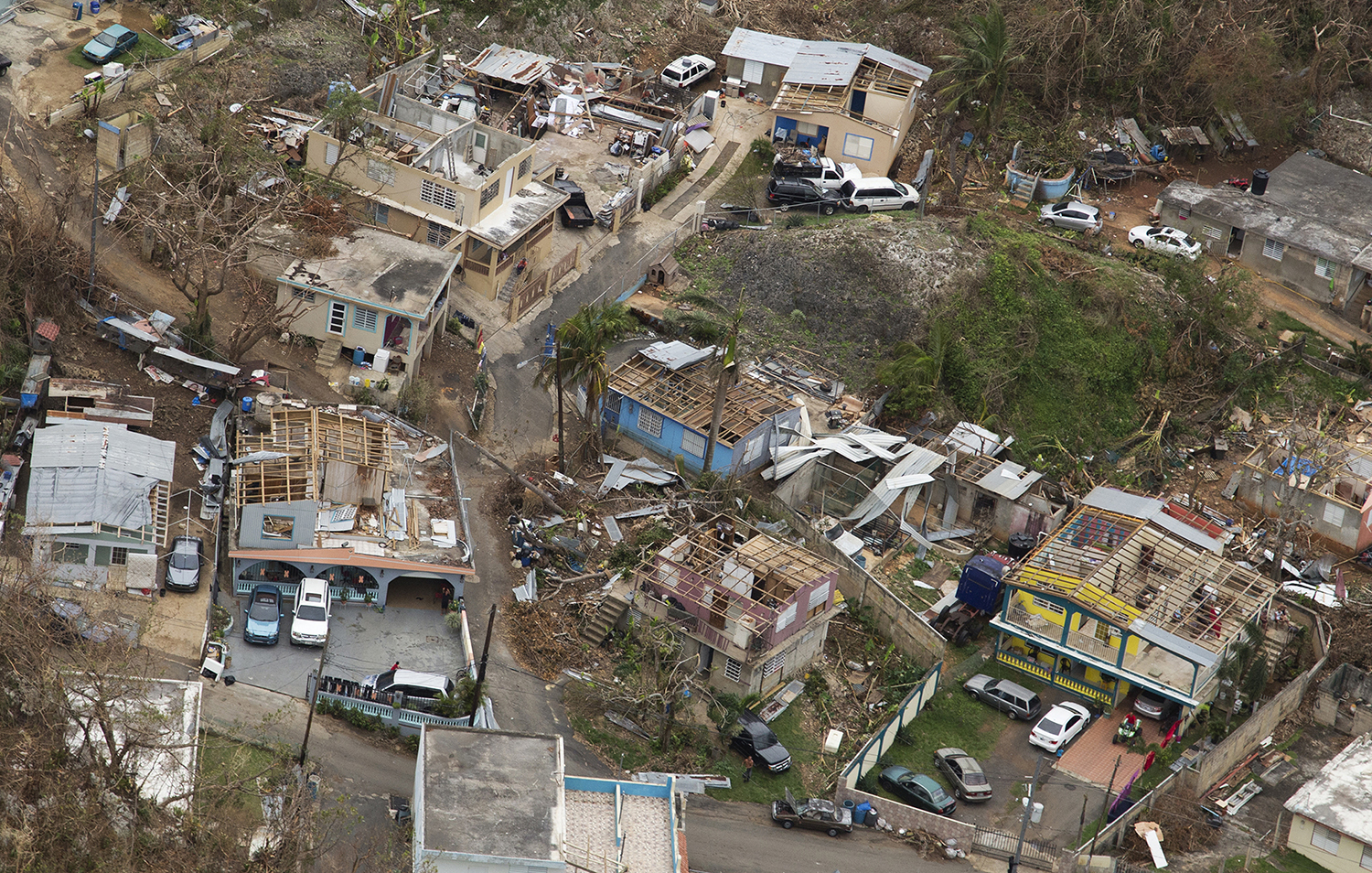The image, captured from an aerial perspective during daylight, depicts the aftermath of a devastating natural disaster, likely a tornado or hurricane. The scene showcases a neighborhood with multiple apartment buildings and houses, many of which have roofs missing, exposing their interiors. Some of these roofs have grids of wood, possibly indicating ongoing construction efforts to repair the damage. The buildings are primarily beige or grey, surrounded by cars in shades of white, grey, and blue, scattered about the area.

The landscape appears to be inclined or sloped, with streets that are unclear and grey, littered with debris. The trees exhibit significant damage, some leafless and others with sparse foliage, and dried plants add to the scene of desolation. Utility poles can also be seen amidst the chaos. Adding to the sense of disrepair, several houses have garages with vehicles parked inside or nearby. Overall, the image portrays an outdoor setting overwhelmed by destruction, with visible damage to infrastructure and the environment.